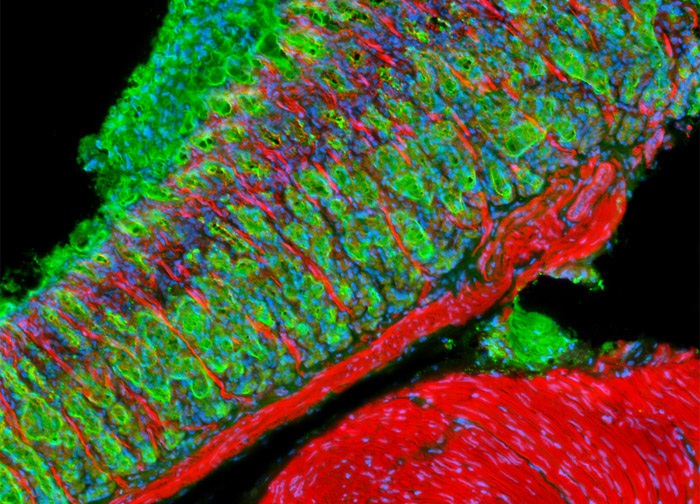The image showcases a highly detailed, abstract representation, likely something viewed under a microscope in a biology lab. Dominated by vibrant greens with striking red accents, the primary subject features an intricate texture reminiscent of scales. These scales span across the center and sides, set against a pitch-black background. Near the bottom, a prominent red blob, resembling blood, contrasts vividly with the green mass above. The picture also includes fleeting touches of blue, orange, and purple streaks, adding depth and complexity to the composition. This compelling blend of colors and forms creates a visually arresting, almost alien-like view, possibly of a cell or microscopic entity, illuminated by varying chemicals or filters.